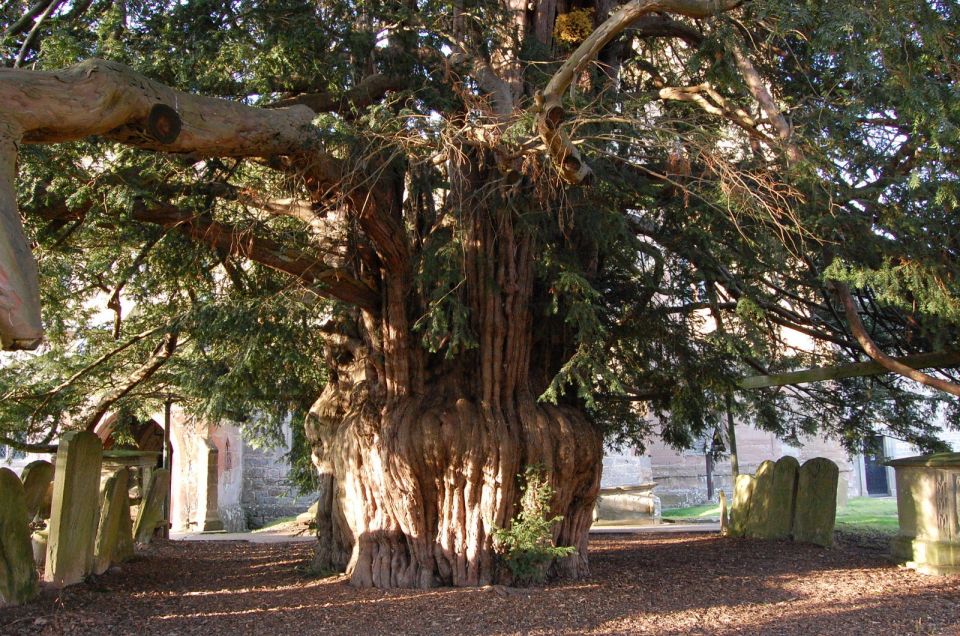In this detailed and realistic photo, the focal point is an ancient and enormous yew tree, potentially hundreds to a thousand years old, situated in the middle of a cemetery beside an old church, possibly in England. The tree is so massive that it dominates the image, although the entire tree isn't fully visible. It features an intricately thick root system that encapsulates its center, resembling a densely packed wooden planter. The expansive trunk, marked with numerous vertical lines and very thick bark, splits into many sections and long limbs, some of which are bare while most are covered in furry green leaves, with a few dead branches hanging. This dense canopy casts a substantial shade over the surrounding area, which is strewn with leaves. Among the roots, a small sapling can be seen growing at the base on the bottom right. Scattered around the tree are old, thin concrete headstones, some of which lean to the side and are overgrown with grass, further emphasizing the age of the cemetery. In the background, partially obscured by the tree, is a building with a visible black door on the right side.